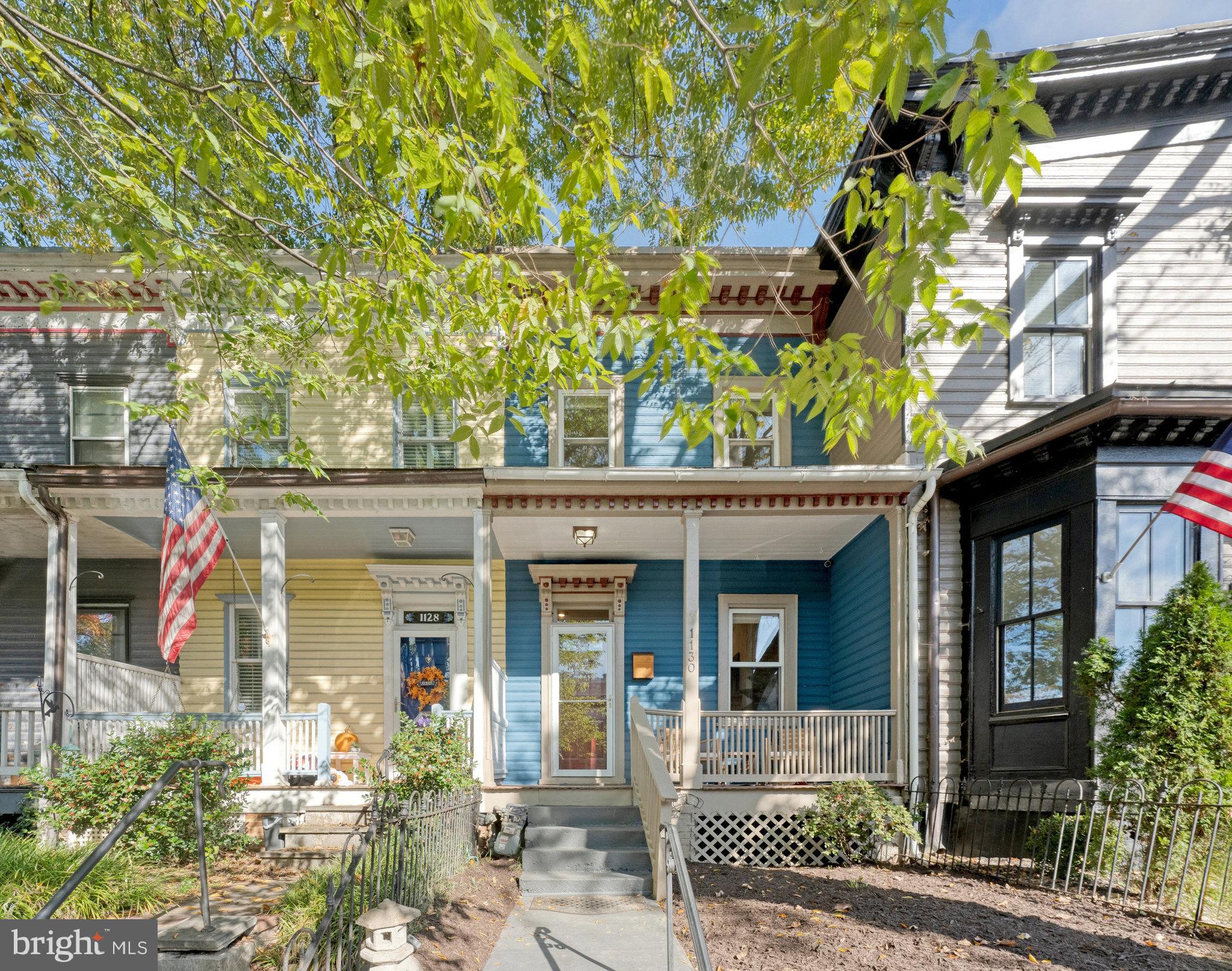The photograph is a detailed and vibrant depiction of a colorful row of two-story homes, each with distinctive features. On the left side, the duplex is painted a cheerful yellow with white trim, adorned with an orange wreath hanging on its blue front door. This unit features three stairs leading down to a small yard filled with green plants and a bush. A prominent American flag is mounted on one of the white columns. Adjacent to it, the bright turquoise duplex mirrors the structure of its yellow neighbor but has a predominantly barren yard with sparse greenery. The larger, partial structure to the right is a white house with a black front screened-in porch, also displaying an American flag. Throughout the scene, detailed wood siding and ornate trims are evident, contributing to the vintage charm of the buildings. The homes are connected by gray steel fences, which define their individual yards, contrasting with the predominantly dirt-covered ground. Concrete pathways guide to the entrances, adding a touch of urban design amidst the rustic atmosphere.